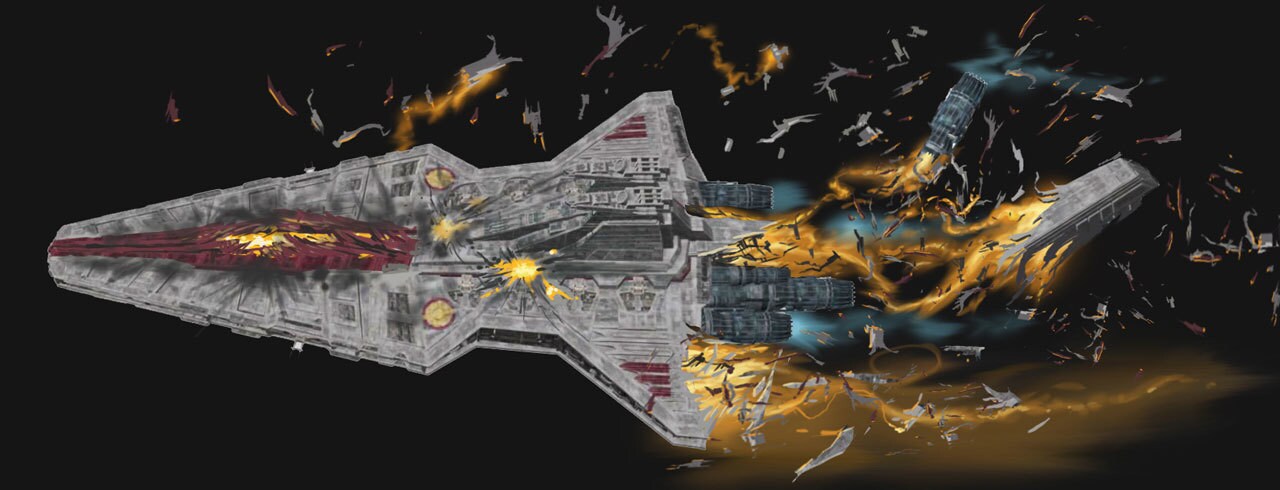The image depicts a futuristic spacecraft set against the stark blackness of outer space, appearing as though it could be a poster or a digital illustration for a science fiction game or movie. The spacecraft, resembling a large arrow with a wide middle section and a narrower end, is primarily gray with white and red markings, including distinctive red lines on the wings and a central red stripe along the front half. The vessel appears severely damaged, with the front section engulfed in flames and the back end violently exploding. Blue flames shoot out from the rear, while orange-yellow flames and fragments of metal erupt from various areas, suggesting an intense, catastrophic event. The scene is chaotic with pieces of the spacecraft flying through the void, giving a dramatic portrayal of destruction in the cold expanse of space.